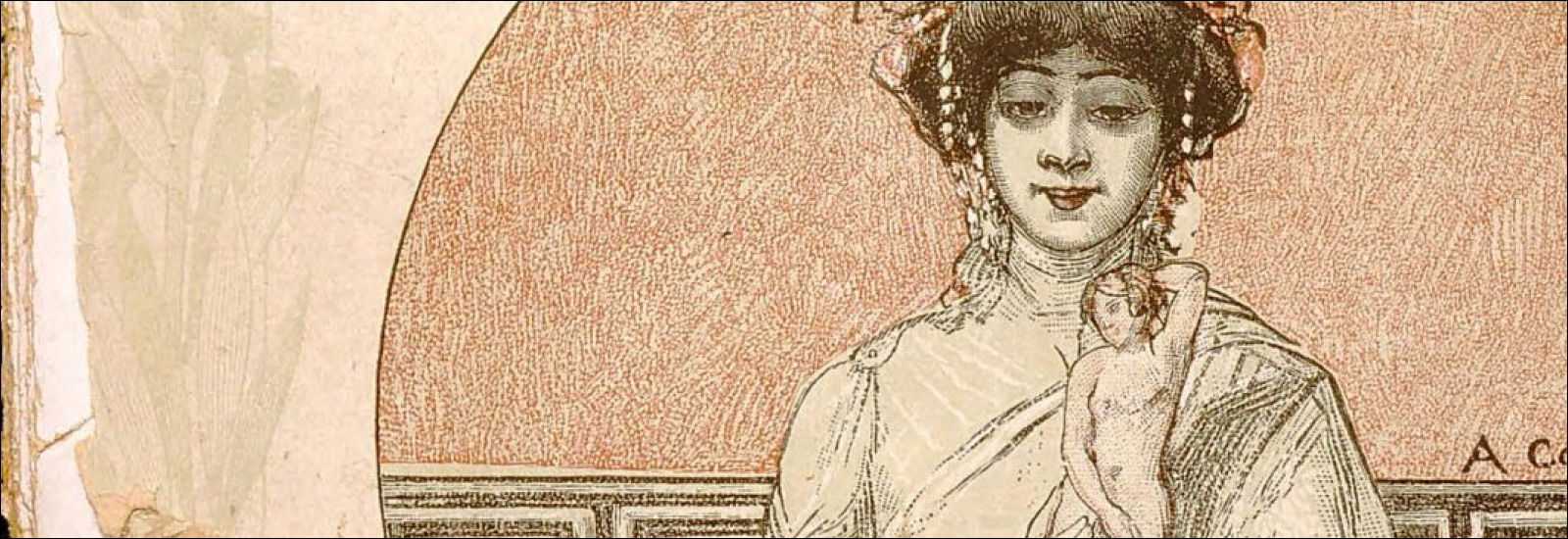The zoomed-in photograph showcases a stylized drawing created with pencil or charcoal, highlighted by a backdrop of red lines randomly overlapping in a crown-like pattern. Dominating the foreground is an image of a woman, adorned in a white dress with her hair elegantly pulled back into an elaborate headdress. She cradles a smaller, nude statue of a woman, which has its arms positioned to cover its head and body, giving an impression of modesty or shyness. The detailed drawing presents both figures in a composition suggestive of an Indian theme, characterized by delicate, pale hues of pink, beige, green, white, and almost black tones. The larger woman’s delicate, small red lips and the intricate fabric draped over her contribute to the rich, textured feel of the artwork, adding to the striking visual intensity of the scene.